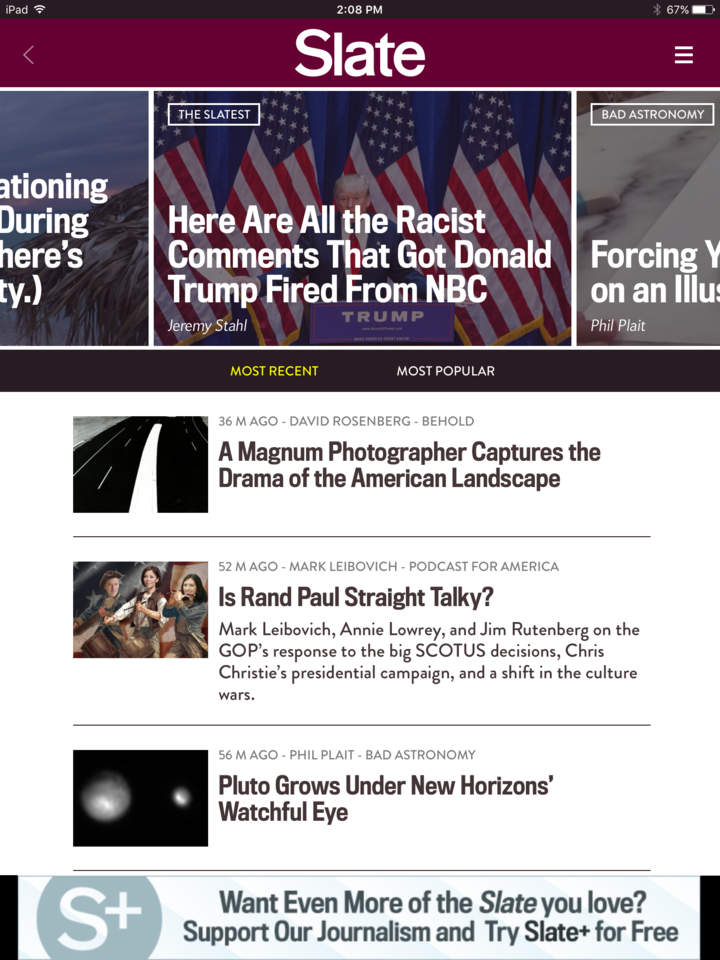The image captures the screen of an iPad displaying the Slate website. At the top of the screen, a thin black bar spans across, showcasing various device indicators. On the left, white text reading "iPad" is accompanied by a signal strength icon. The center of this bar displays the time, "2:08 PM," also in white text. To the right, the bar indicates that Bluetooth is on and the battery level is at 67%, represented by a horizontal battery icon.

Beneath this, a maroon panel stretches across the top portion of the screen. In the center of this maroon panel, "Slate" is written prominently in large white letters. Below this, a large rectangular section occupies the majority of the screen's real estate. This section features a background of flags and an image of Donald Trump, with overlaid white text reading, "Here are all the racist comments that got Donald Trump fired from NBC."

Flanking this central rectangle are two partially visible panels, each with distinct backgrounds and text. The one on the right has a small box in its top-left corner labeled "Bad Astronomy." The middle section of the panel sports a box labeled "The Slatest."

A black band runs below these panels, offering navigational options. "Most Recent" is clickable in yellow letters, and "Most Popular" is clickable in white letters. Below this navigation band are three clickable article thumbnails, each set against a white background with black text. The articles are titled: "A Magnum Photographer Captures the Drama of the American Landscape," "Rand Paul Straight Talkie," and "Pluto Grows Under New Horizons Watchful Eyes." Each article boasts a thumbnail image to its left, details about the posting time, author names, and a brief description for the Rand Paul article.

At the bottom of the page, a light gray banner invites further engagement with the text: "Want even more of Slate you love? Support our journalism and try Slate Plus for free." To the left of this text is a darker gray circle containing a white "S" and a plus sign.